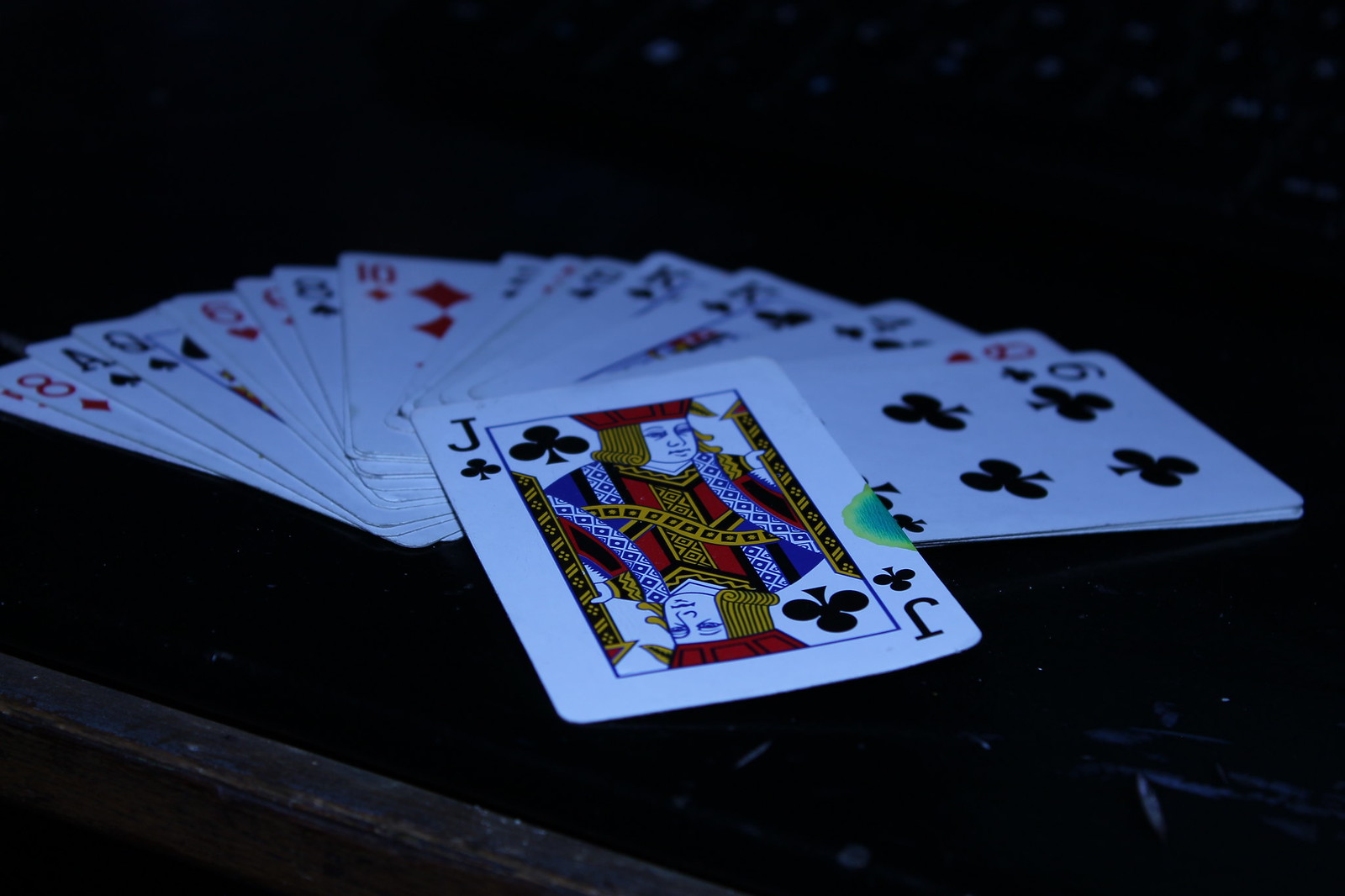In the image, a dark wooden tabletop emerges from a very dark background, punctuated with identifiable scratches and marks on the lower right corner. The edge of this table is visible towards the lower left corner, providing a rough and rustic charm. At the center of this setting, a close-up view reveals a fan of playing cards arranged in a semi-circle. The spread includes various suits and numbers: beginning from the left, there is an eight of diamonds, a spade, a queen, a six of hearts, a ten of diamonds, and extending to a six of clubs on the far right. Notably, in the heart of the fan lies a joker of clubs, prominently facing upwards. This particular joker card reveals an intriguing detail—a bluish-green watercolor stain on its edge, adding an element of mystery and character to the otherwise pristine deck.